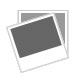The image captures a sleek kitchen counter made of multi-shaded gray marble granite, which extends elegantly up to a white tiled wall. There are two coffee mugs—one decorated with crisscross black and white designs and the other with linked circles—each resting on matching saucers. Between them sits a small container resembling a soufflé cup, filled with what appear to be butter pots. In the background, three glasses of water are visible. Adorning the wall are black decorative elements, including a pineapple, a kettle pouring tea into a cup, a heart, and utensils (fork, spoon, and knife). Above these are the words "kitchen" and "coffee," artistically integrated into the decor against the pristine white tiles.